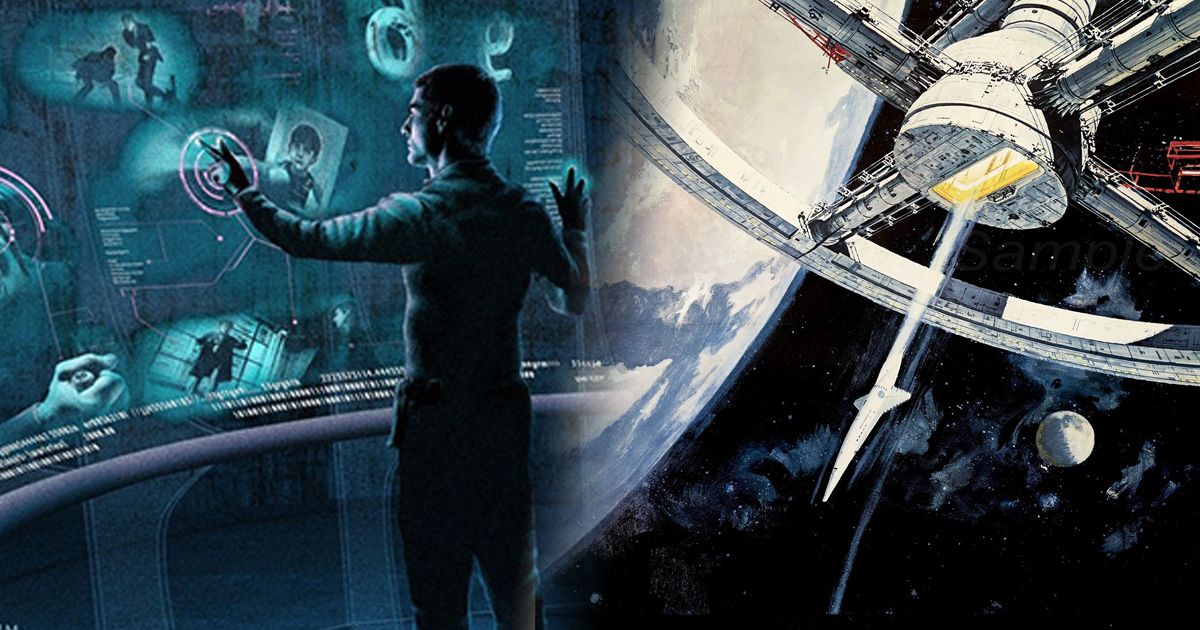This vivid, horizontally elongated digital artwork merges elements of science fiction and surveillance, creating a compelling scene. The left side of the piece features a man with close-cropped hair, situated in a futuristic space laboratory. He stands in three-quarter profile, intently manipulating a large, curved digital display screen reminiscent of the technology from "Minority Report." The man, depicted from head to just below his knees, is shrouded in dark clothing, blending into the shadows. The screen he interacts with shows various images, including security camera feeds, photographs of individuals, and small, illegible text, all rendered in shades of gray and blue.

Transitioning to the right half of the image, the interior view dissolves into the vastness of outer space. A dark, bluish cosmos serves as the backdrop for an imposing space station designed as a circle intersected by an X, highlighted by touches of bright yellow lights. This space station hovers near the corner of a planet that bears a striking resemblance to Earth, accompanied by a distant moon.

The overall color palette of the artwork features predominant dark blues with mysterious undertones, punctuated by bright, luminous highlights that add depth and intrigue to the scene.